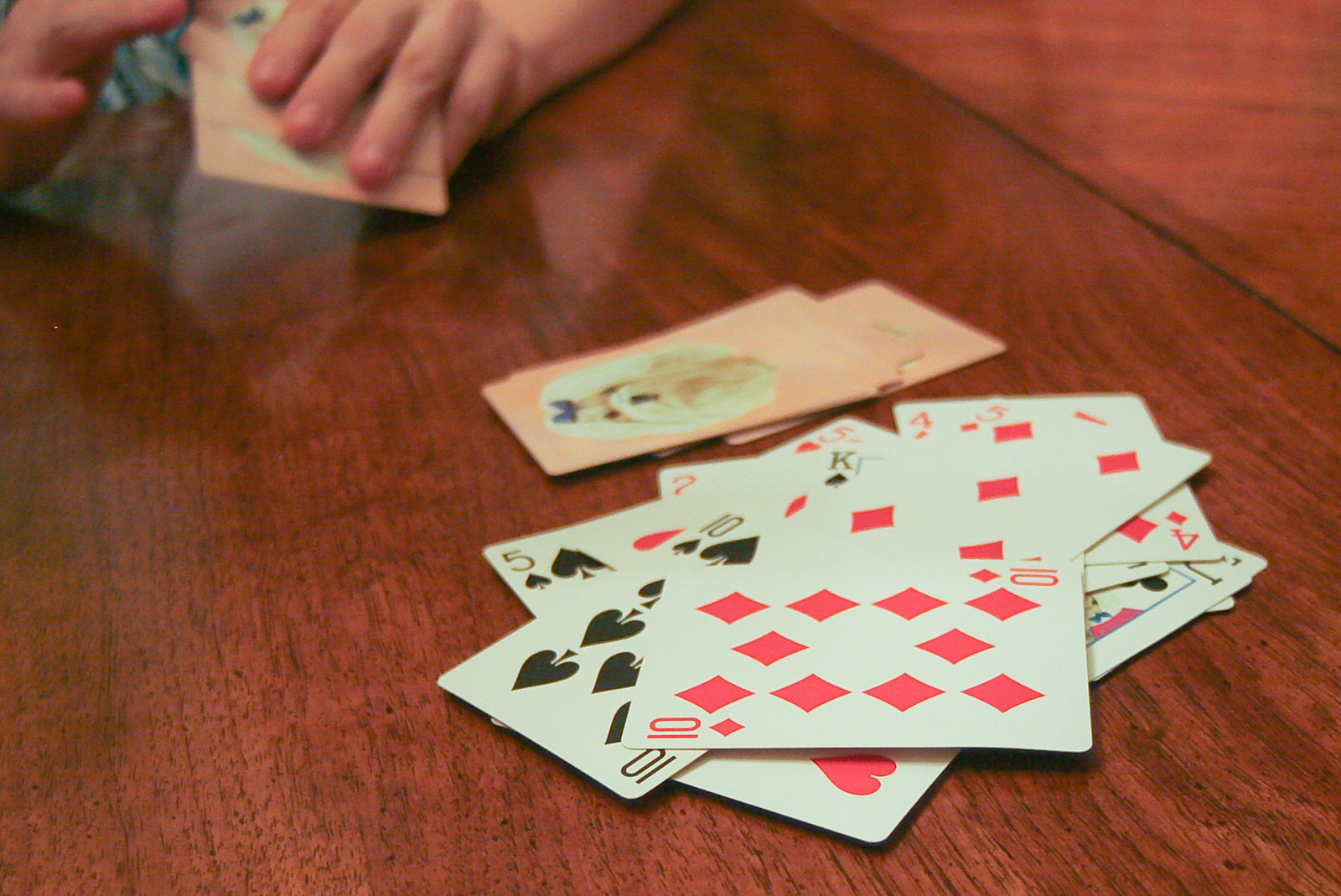In the foreground of the image, a set of playing cards is scattered on a varnished wooden table, some positioned face up and others face down. The table’s clear, reflective finish allows light to glint off its surface, accentuating the grain of the wood, which runs diagonally from the bottom right to the upper left of the image. A person's left hand, holding a few cards, is partially visible, accompanied by a glimpse of their right hand and the fabric of their clothing. The clothing features a blend of light and dark blues, white, and tan colors. Some of the playing cards show typical suits such as diamonds, clubs, and spades. The decorative backs of the cards display a light pink or tan hue with circular patterns. In the background, blue shoes and the person's legs, draped in cloth, are faintly visible, contributing additional context to the scene. The image is sharply focused, providing a detailed and coherent view of the setting and the figure involved.